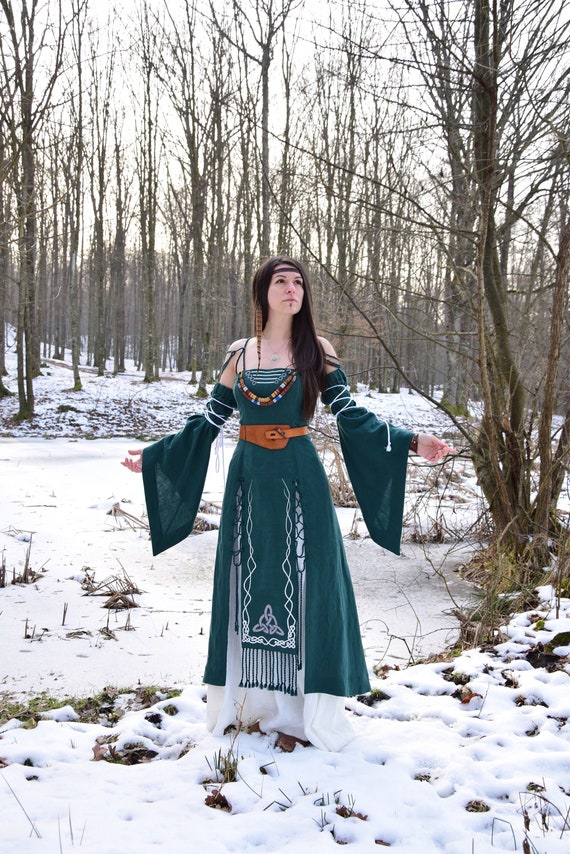This photograph captures a striking image of a young woman standing in a snow-covered, barren forest, evocatively blending elements of Native American and medieval Celtic aesthetics. The woman, who has long, waist-length dark hair draped over one shoulder, wears a thin, dark leather headband adorned with a long, brown feather. Her face features a mark on her chin reminiscent of traditional Native American tattoos. 

Her attire is an aqua-colored, Celtic medieval-style dress that might resemble a wedding gown. The dress has delicate spaghetti straps and separate, billowy sleeves that are only attached by elastic bands around her upper arms, tied with white cords. The garment also includes a decorative, red belt and an apron-like front panel adorned with white fringes, dropping to ankle length with a glimpse of white lace underneath. Complementing her outfit is a necklace featuring a turquoise stone set in silver, adding a touch of elegance.

The woman stands barefoot with her arms outstretched, her long, baggy sleeves draping gracefully over her forearms. The surrounding landscape, with a frozen pond and leafless trees, adds to the serene and somewhat mystical winter setting, imbuing the photograph with a sense of historical and cultural fusion.